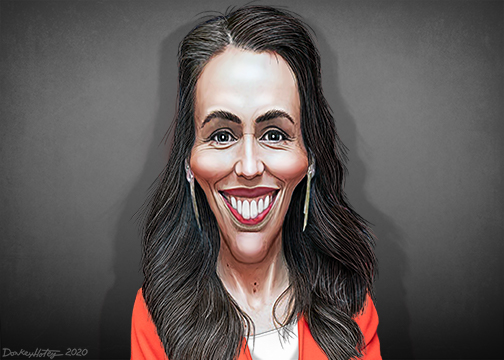The image features a digitally created, slightly realistic caricature of a woman, possibly a political figure, characterized by exaggerated facial features. Her head is disproportionately large, reminiscent of a bobble head, adorned with very long black hair and sharp, made-up eyebrows. Her eyes are encircled with wrinkles, and her cheeks are noticeably blushed. She wears striking red lipstick. The woman is clad in an orange dress paired with a white undershirt and dons long earrings.

Her facial proportions are markedly off, with a particularly large forehead, highly pronounced cheekbones, and disturbingly huge, white teeth that give her an almost grotesque appearance. Her chin resembles the shape of a golf ball. The background is a uniform gray, enhancing the focus on her detailed, caricatured visage.

At the bottom left of the image is a watermark of the artist's signature, which appears to read "Don Quixote Incursive 2020." The artwork cuts off at the chest, making it more of a headshot or bust, though her position (sitting or standing) is ambiguous. The overall color palette includes shades of coral, black, red, and various grays, contributing to the cartoonish, digitally-rendered style of the image.